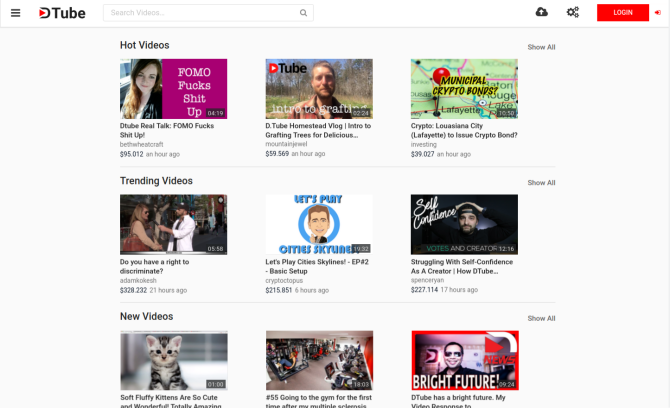The image depicts an alternative YouTube site called Dtube, characterized by a white background with predominantly black text. 

In the top left corner, there's a logo featuring the word "Dtube" with a red arrow forming the "D" and the remaining letters in black. In the top right, there are a search box, a cloud icon, a gears icon, and a red login button.

Below the header, there are three categories of videos arranged in three rows of three thumbnails each. The first category is "Hot Videos" which include:
1. A young girl's head with text "Dtube Real Talk: Fomo Fucks Shit Up."
2. A man's head against a forest background with the text "Dtube Homestead Vlog: Intro to Grafting Trees Were Delicious."
3. A pin on a map with the text "Crypto Louisiana: City Lafayette to Issue a Crypto Bond."

The second category is "Trending Videos" featuring:
1. A man talking to a woman with the text "Do You Have a Right to Discriminate?"
2. A man's cartoon head in a blue circle with the text "Let's Play City Skylines."
3. A man with hands over his head against a black background with "Self Confidence" written in white, accompanied by the text "Struggling with Self Confidence as a Creator. How Dtube."

The third category is "New Videos," showing:
1. An image of a kitten with text "Soft Fluffy Kittens are So Cute and Wonderful."
2. A picture of a gym with partially obscured text starting with "Going to the Gym for the First Time After my Multiple Sclerosis..."
3. A man's head with "Bright Future" written in white and the text "Dtube Has a Bright Future: My Video Testimony to..."

Overall, Dtube appears to be a YouTube alternative streaming service showcasing diverse content ranging from personal vlogs and self-improvement talks to gaming and cryptocurrency discussions.